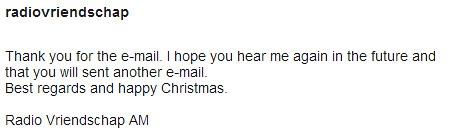The image displays a simple, typed response to an email on a white background with black text. At the top, in bold and darker black lettering, it reads "Radio V-R-I-E-N-D-S-C-H-A-P," which may suggest an internet radio station, although the exact meaning is unclear. The message beneath begins with "Thank you for your email," followed by a hopeful note about future interactions: "I hope you hear me again in the future and that you will send another email." The sender extends well wishes with "Best regards and happy Christmas." At the bottom left, the text concludes with "Radio V-R-I-E-N-D-S-C-H-A-P-A-M."